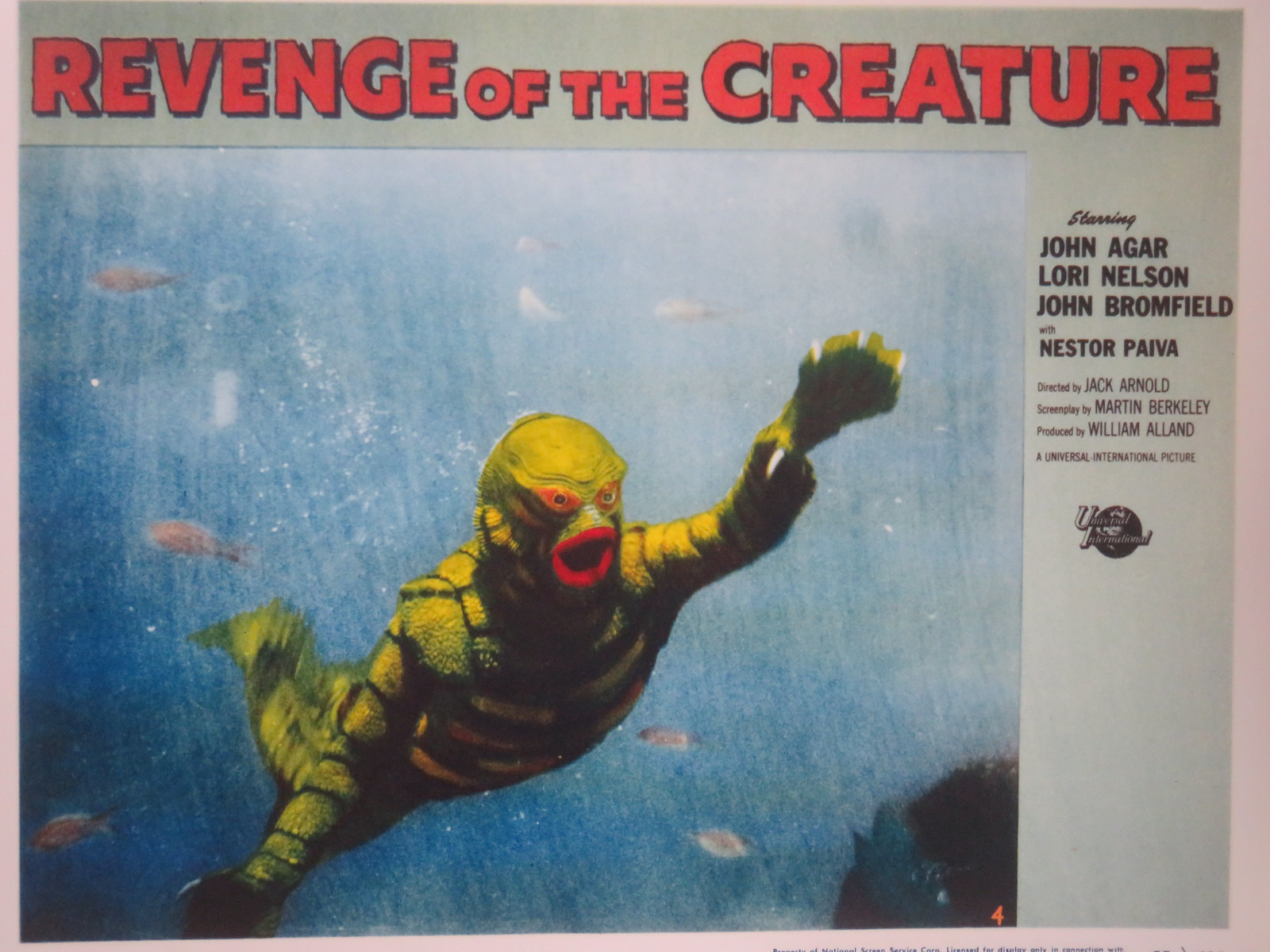The promotional image for the movie "Revenge of the Creature" features the film title prominently printed in bold, red capital letters. Beneath the title, an underwater scene unfolds, showcasing a monstrous green creature with a body marked by dark green lines and patterns. The creature's face is striking, with outer eyes lined in red and black eyeballs, and an open, large red mouth. The eerie aquatic environment is blue, populated by various white and pink fish swimming around the creature, giving the impression it is deep in the ocean. To the right side of the image, in black text, the cast is listed, highlighting John Agar, Lori Nelson, and John Bromfield with Nestor Paiva. The same section includes credits for the director, screenplay, and other production details in a smaller font. The overall scene captures the otherworldly and menacing aura of the creature, as well as the film's undersea setting.